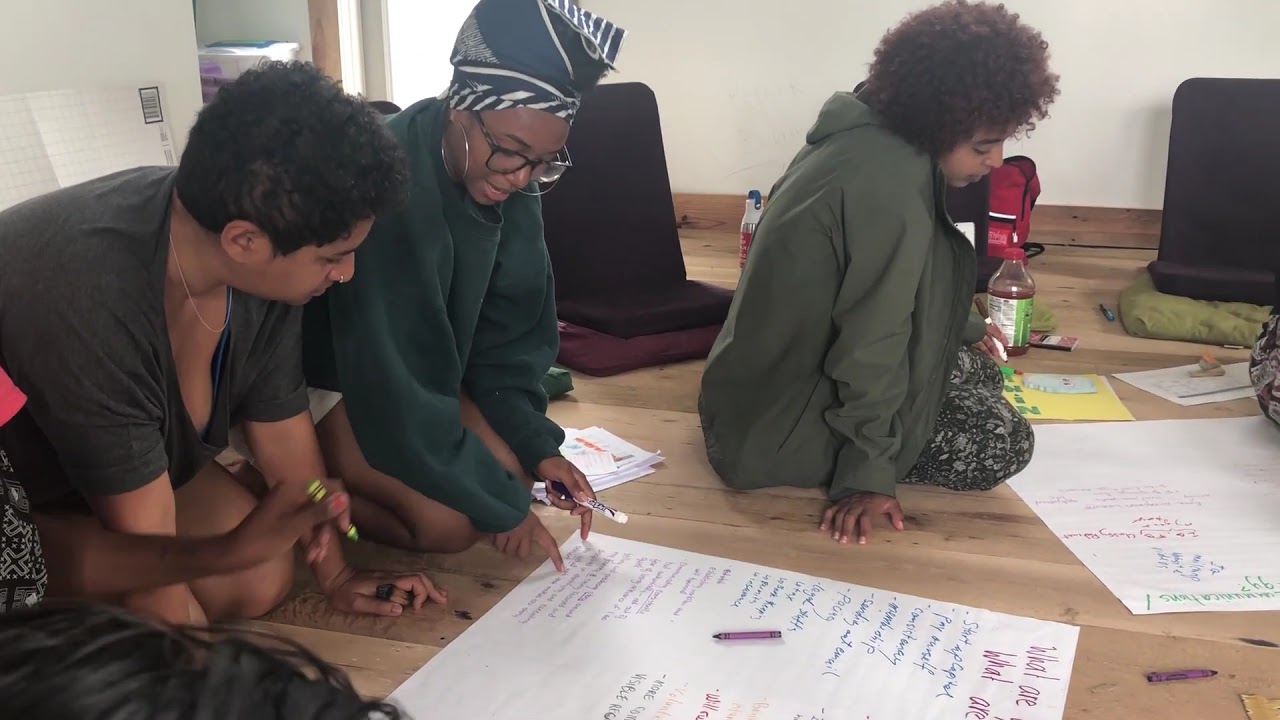The image depicts a group of young people of color, likely older teenagers or college-aged, engaged in a collaborative project. They are gathered on a wooden floor adorned with white posters, markers, and crayons, deeply immersed in brainstorming and writing. The setting appears to be a classroom with white walls and wooden flooring, featuring scattered cushions and occasional visible backpacks. The individuals, consisting of predominantly young women and one person of indeterminate gender with short hair, are clad in earthy tones such as dark green, moss, and gray attire. Among them is a young woman with glasses, large hoop earrings, and her hair wrapped in a scarf; another with shorter curly hair; and a person with dark black hair in a dark green t-shirt. They are intently discussing and mapping out concepts on the posters, some of which contain words like "start AP Capital," "pay our self," "consistency," and "ownership." The scene captures a moment of focused collaboration and creative expression.